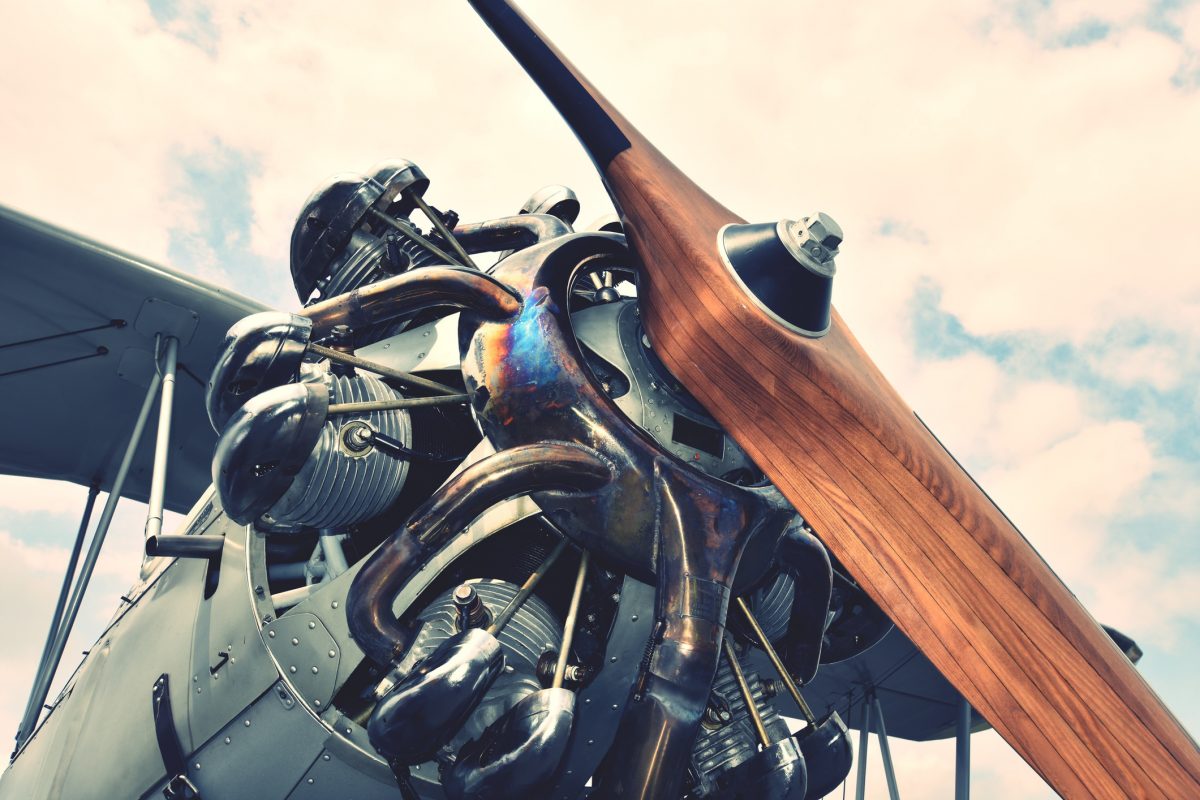The rectangular image, approximately six inches wide by four inches high, captures an angled upward view of the front propeller of a single-passenger or two-seater airplane. The wooden propeller, which is brown, extends diagonally toward the lower right-hand corner, narrowing and turning black as it extends off the screen. The propeller's center features a black conical cap with a silver nut on the end. To the left, the exposed engine components, which have a tarnished metal appearance showing oil discoloration—blue, purple, and yellow hues—are visible, including several identical units with sandwiched metal discs at their bases and shiny black, canoe-shaped elements on top. The plane’s underbelly, a light gray color, and the dark gray underside of its wings can be seen in part. The background is a mostly cloudy sky with patches of blue peeking through, lending a bright, natural atmosphere to the scene. The image could be a realistic painting or a highly detailed computer-generated art piece.